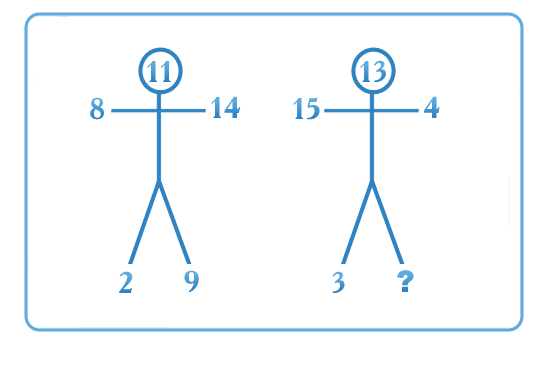This image is a detailed diagram drawn in turquoise blue against a white background. The overall shape of the diagram is oblong. On the left side, there's a circle containing the number 11. Below the circle, a structure resembling a stick figure is depicted. This figure includes a crossbar with the number 8 on its left and the number 14 on its right. Below this crossbar, there's a vertical line leading to two more lines extending horizontally, enhancing the stick-figure resemblance. The line on the left of this vertical extension is labeled with the number 2, while the line on the right is labeled with the number 9.

On the right side of the diagram, a similar figure is shown. At the top of this figure, a circle encloses the number 13. Below this circle, parallel numbers 15 and 4 appear on the left and right sides of the horizontal crossbar, respectively. Continuing downward, on the left of the lower vertical line is the number 3, whereas the right side intriguingly features a question mark instead of a number.

This detailed diagram highlights numerical labels and complex stick-figure-like formations, suggesting an abstract or conceptual illustration.